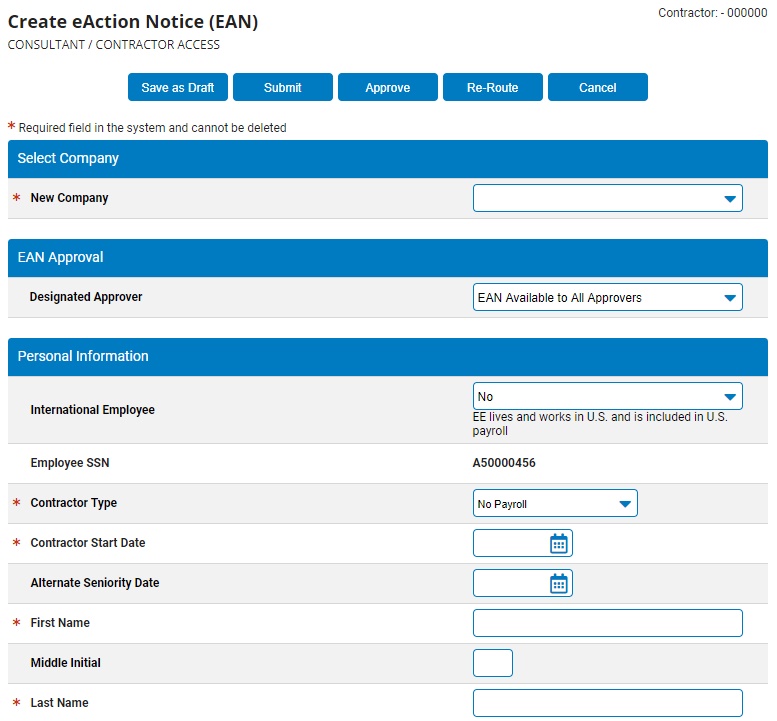The image displays a detailed form interface for creating an "e-Action Notice" (EAN) in a contractor management system. In the top right corner, the form is marked with "Contractor-0000". There are several action buttons including "Save as Draft," "Submit," "Approve," "Reroute," and "Cancel." Users are prompted to select a company from a drop-down list next to the field labeled "New Company."

The form further includes sections for "EAN Approval," asking for the "Designated Approver" with an adjacent field showing "EAN available to all approvers." The "Personal Information" section indicates that the individual is an "International Employee," with a field stating "No" under this label. The form specifies that the employee "leaves and works in the U.S. and is included in U.S. payroll." The employee’s SSN is listed as A50000456.

Additional fields capture information about the contractor, including:
- Contractor Type: No Payroll
- Contractor Start Date
- Alternate Service
- Seniority Dates
- First Name
- Middle Initial
- Last Name